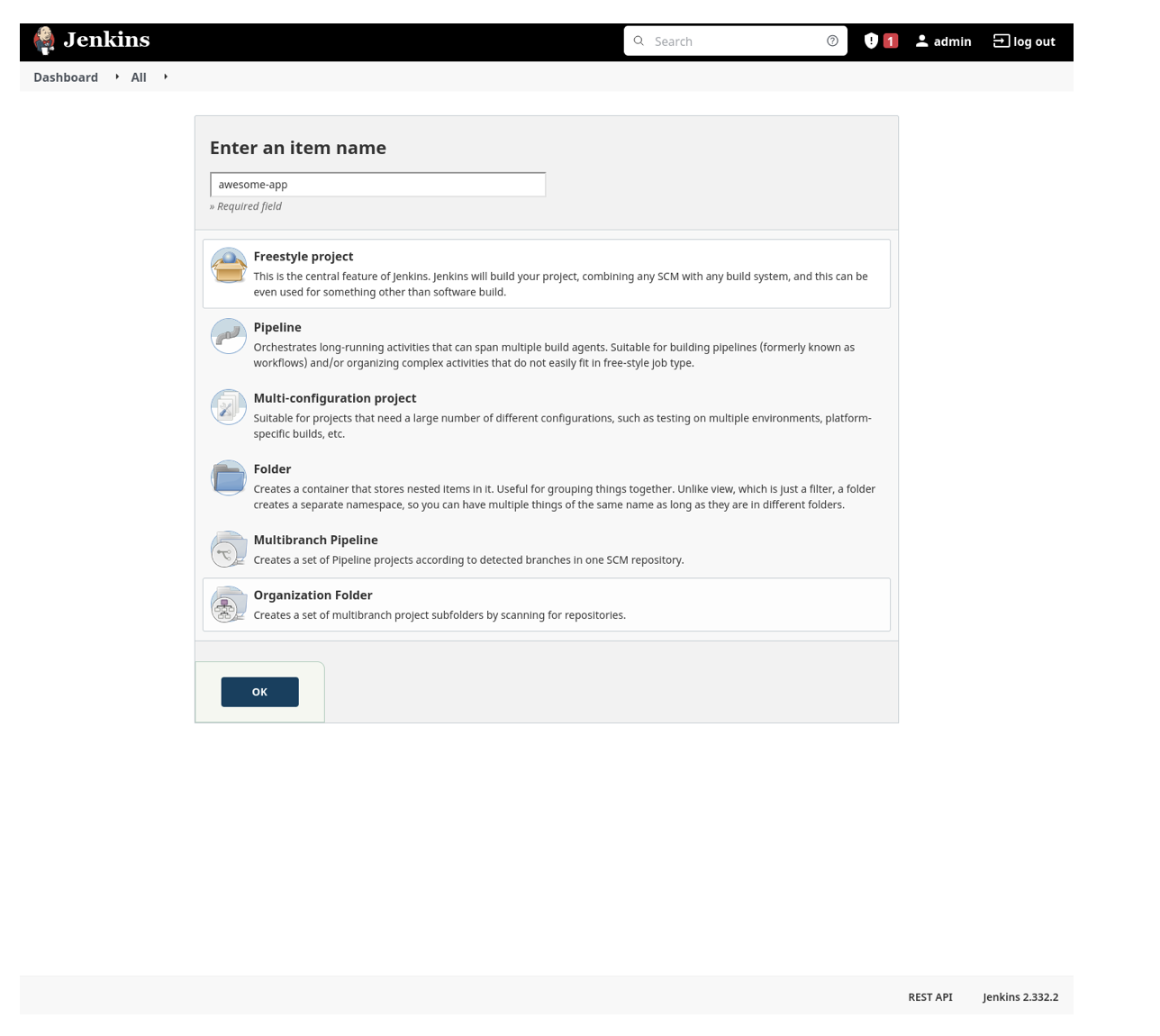The top part of the interface features a black-and-white header that reads "Jenkins." Inside the header, there is a white search box with the text "search" in gray and an icon resembling a shield with an exclamation point inside it. Next to this is a red square with a white number "1" and the word "admit." To the right, there's an option labeled "log out."

Below the header is a gray navigation pane. In a darker shade of gray, it displays options such as "dashboard" and "all."

The main background of the interface is white. Centered within this is a gray square. At the top of this gray square, black text reads "Enter an item name." Below this is a white rectangle resembling a search box, with the phrase "awesome-dash-app" typed into it. Directly beneath the search box, "required field" is indicated.

Further down, there is another white rectangle containing the text "freestyle project" in black. This section elaborates that "This is a central feature of Jenkins. Jenkins will build your project on any SCM with any build system and can even be used for projects other than software builds."

Underneath, the interface displays several options in gray text: "pipeline," "multi-configuration project," "folder," and "multi-branch pipeline." Each has a brief description:
- "Pipeline": Suitable for projects with a large number of different configurations, such as testing on multiple environments, platforms, specific builds, etc.
- "Multi-Branch Pipeline": Creates a set of pipeline projects according to detected branches within a single SCM repository.

Lastly, a white rectangle reads "organization folder," with the description: "Creates a set of multi-branch project subfolders by scanning for repositories."